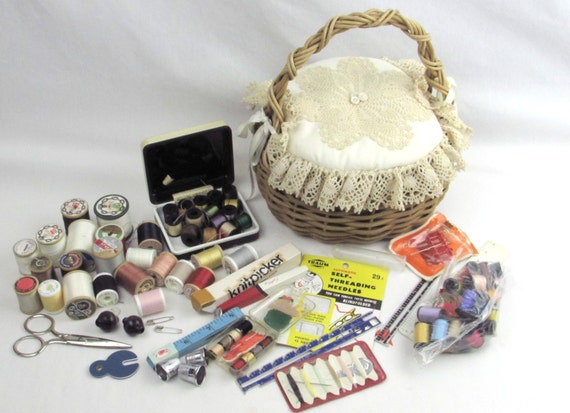The image showcases a detailed collection of sewing notions meticulously arranged on a white sheet. Dominating the left side, there is an assortment of spools of thread in various colors, including white, yellow, dark rose pink, regular pink, coral, red, gray, black, green, and purple. These spools range from medium-sized to tiny ones, including even tinier bobbin spools. Next to this array is a small open case filled with minuscule baby spools with black plastic centers. A silver pair of scissors lies close by, alongside self-threading needles, safety pins, and thimbles—three silver ones. Additional sewing tools include a tape measure, small rulers, a knit picker, and needles. At the top, there's a tan woven basket with a handle, featuring a lacy, white pillow that might serve as a pin cushion. The pillow is adorned with a lace flower on the front and lace trim around the edges, secured to the basket with white ribbons. The overall presentation of these sewing supplies conveys a sense of organization and preparedness for intricate sewing tasks.